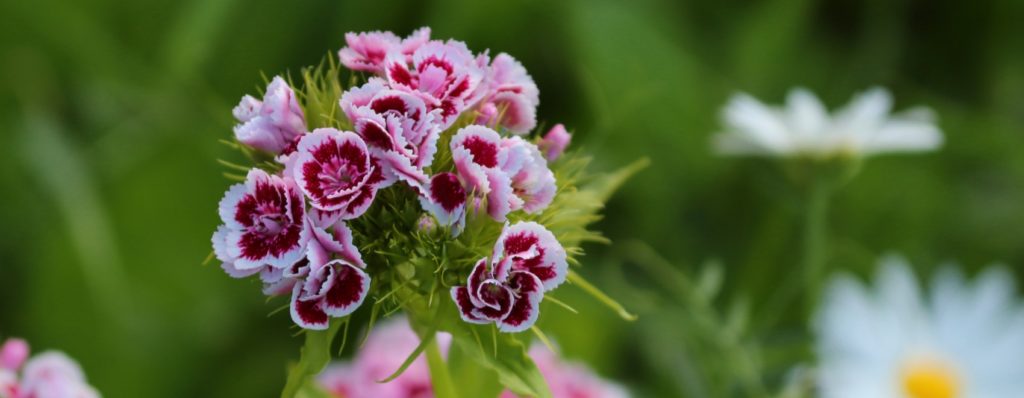This vibrant color photograph captures a close-up of a multicolored flower set slightly off-center to the left. The focal flower displays a stunning gradient of hues, transitioning from white-tipped petals to a deep burgundy, and finally to a soft pink towards the center. Its inner part features a bunch of green, pointy leaves. Below this main flower, nestled just underneath, is another pink bloom, adding layers to the foreground. In the lower left corner of the image, there's an additional pink flower, while the bottom right corner showcases two white daisies with yellow centers, adding a charming contrast.

The background, blurred to emphasize the focal flowers, is a rich tapestry of greens and additional foliage, suggesting the setting is either a lush garden or a wild, natural habitat bathed in sunlight. Despite the lack of text, the image communicates a serene and vibrant spring or summer day, with the blurred greenery hinting at a dense array of plant life. The colors, primarily various shades of green alongside pink, purple, yellow, and white, contribute to a lively and inviting scene.